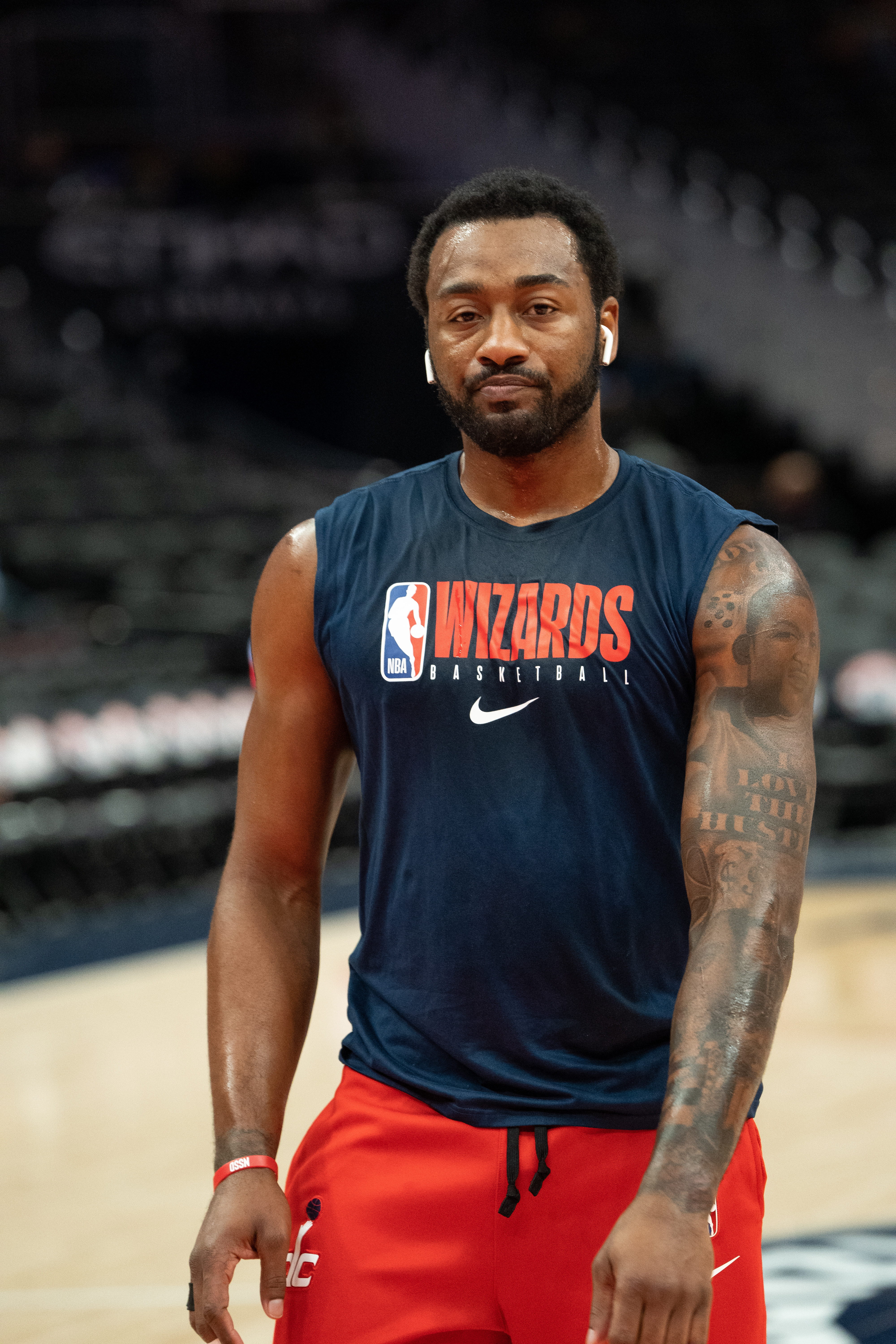The image features an African-American basketball player on what appears to be a practice or pregame session. He stands in the center with a backdrop of a blurred basketball court and audience stands, accentuating the focus on him. The player has short black hair, a mustache, and a beard, and he wears white AirPods in his ears. His expression is serious and unsmiling as he looks straight ahead. 

He is dressed in a navy blue sleeveless tank top with "WIZARDS" in bold red letters and "BASKETBALL" in white beneath, alongside a Nike swoosh and the NBA logo. His entire right arm is adorned with prominent tattoos, including one that reads "I love the hustle." His muscular build is evident through the sleeveless shirt. Additionally, he wears red shorts featuring the DC logo of the Washington Wizards.

The blurry background of the light brown wooden court and black seating area suggests a pregame or practice atmosphere, further emphasizing the clear, detailed depiction of the athlete. A bronze bangle is also noticeable on his right arm.